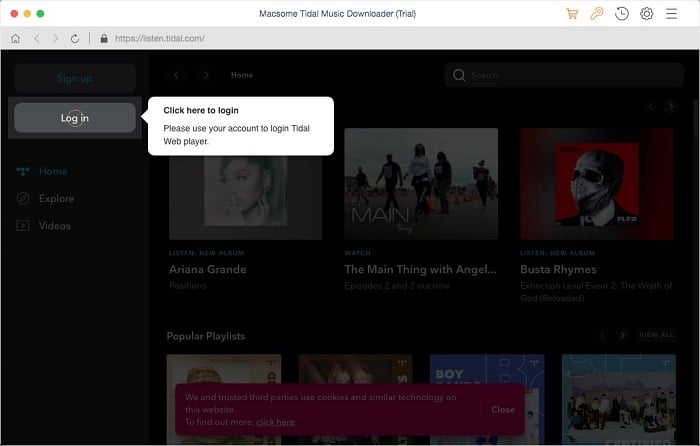This image appears to be a screenshot of a music application interface, likely from a web player called "Tidal." The background contains various icons and pictures indicative of a playlist setup, but the details are obscured due to a prominent log-in prompt. At the top of the screen, the application is labeled "Maxim Tidal Music Downloader Trial," with three buttons in red, yellow, and green positioned nearby.

In the center of the image, a white and gray pop-up window is displayed. This window features a log-in button shaped as a long, skinny rectangle with curved ends, containing the text "Log In" in white. Adjacent to this button, a speech bubble with the text "Click here to log in" protrudes to the right. Below this instruction, additional text reads, "Please use your account to log in," accompanied by the descriptive title, "Web Player." The topmost section of the screen includes the URL "listen.tidal.com," while the rest of the screen content remains indistinct due to blurriness.